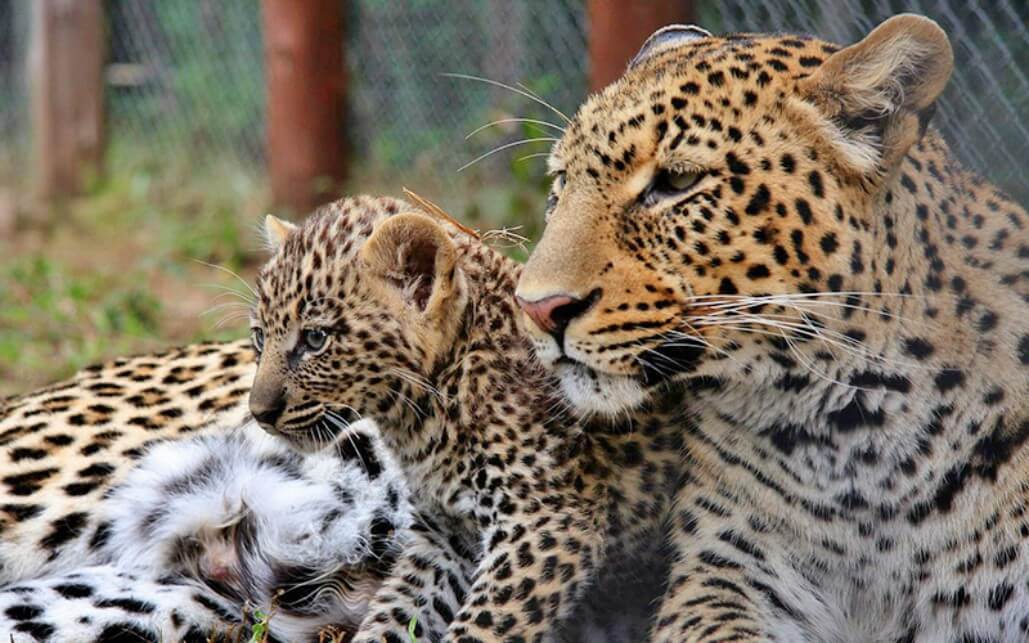This professionally taken nature photograph captures a serene scene of cheetahs in captivity. Dominating the foreground is an adult cheetah with a pink nose, long white whiskers, and striking yellowish-tan fur, lavishly dotted with black and brown spots. She gazes off to the left, her ears slightly laid back. Nestled beside her is her smaller offspring, also adorned with dark spots and exhibiting vivid green eyes, mirroring her posture and gaze. Partially visible, another cheetah's belly with white fur and spots lies to their left, suggesting a protective or relaxing posture. The blurry background features the steel posts of a double-layer chain link fence and a patch of brown and green grass on the left, completing this intimate glimpse into their enclosed habitat.